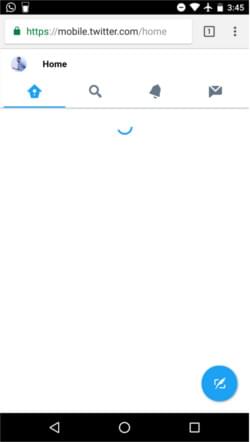A screenshot displays an Android phone with an open web browser, likely Chrome, showing the mobile version of Twitter. The URL reads mobile.twitter.com. The page is currently in the process of loading, displaying a static screen with minimal content. At the top of the page, the user is signed into their Twitter account, as indicated by the visible profile icon.

The interface comprises four icons representing different sections: Home, Search, Alerts, and Messages, with the Home icon being highlighted. A "Create Post" button, depicted as a small box with a quill inside, is situated at the bottom right corner of the screen.

The browser has only one open tab, as indicated by the tab management area. The device's time display shows 3:45, and the status bar reveals the phone is in airplane mode, likely causing the page's failure to load as airplane mode disables all wireless connections.